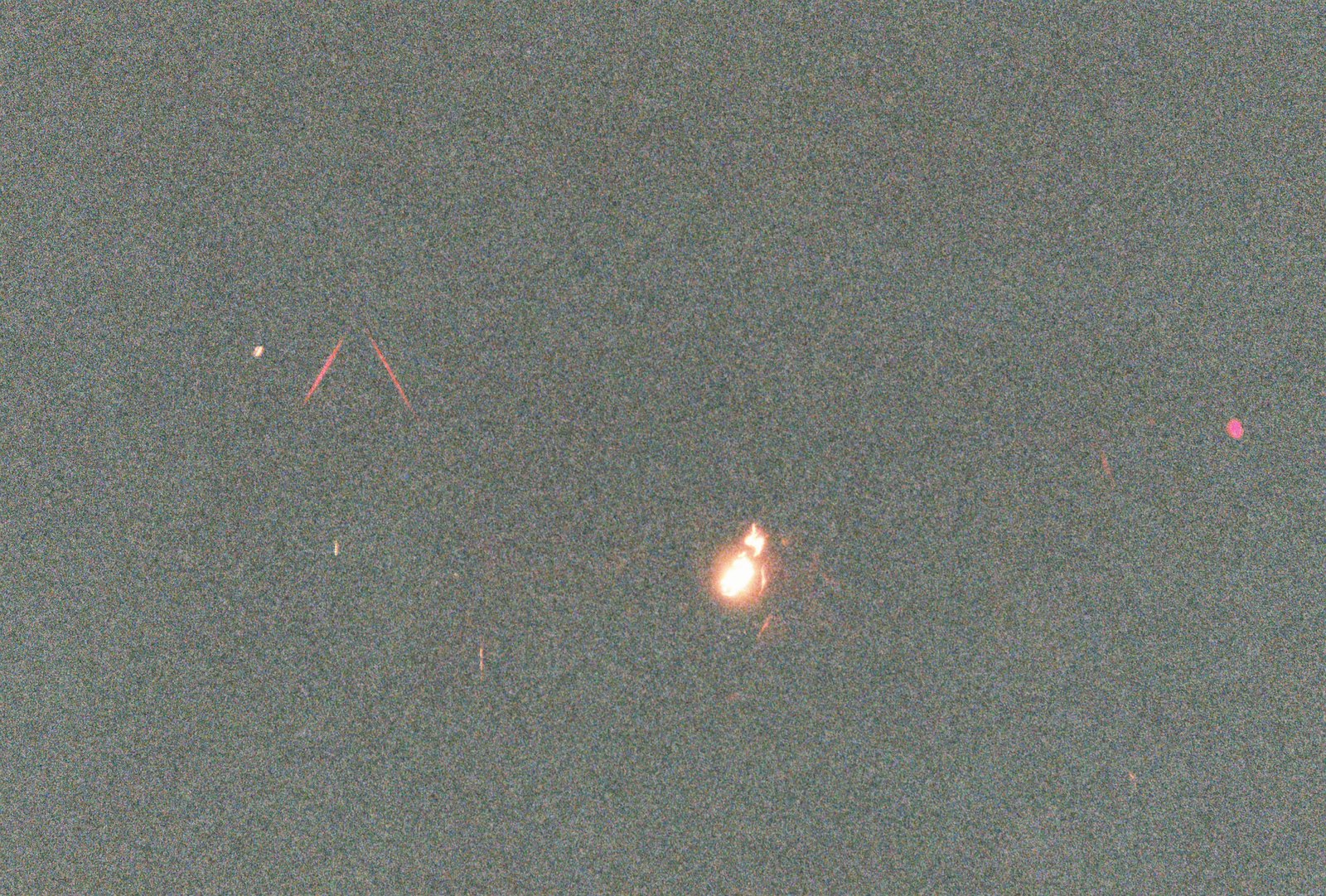This grainy, staticky photograph displays a predominantly gray and black background that spans the entire frame. It appears to capture a night sky filled with numerous specks and dots of gray, black, and white. Centrally placed is an eye-catching orange glow resembling a flame, with an oval shape and a diamond-like fiery tip at the top, radiating an orange and reddish hue. To its left, there are two distinct red or pink diagonal streaks, one veering left and the other right, accompanied by two small white specks. The right side of the image features a single bright red, almost orb-like, non-circular dot. An additional pink dot is also visible towards the right. Throughout the image, subtle streaks and flecks of red are interspersed, adding vibrancy to the otherwise hazy, staticky, and predominantly monochromatic composition.